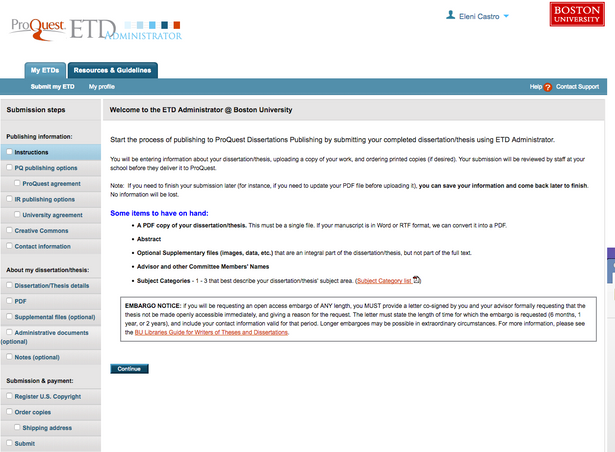**Detailed Caption:**

This image showcases a computer screen displaying the ProQuest ETD (Electronic Theses and Dissertations) Administrator interface, specifically for Boston University. The interface is designed to assist users in the process of submitting their dissertations for publication through ProQuest Dissertations Publishing. 

On the left-hand side of the screen, there's a gray box titled "Submission Steps," providing a step-by-step guide for the submission process. Adjacent to this, a teal box offers "Publishing Information" and "Instructions" related to the submission. The screen lists various segments that users need to complete, including:

- ETDs and resource guidelines
- Submission steps
- Publishing options, which includes choices like ProQuest Agreement, IR Publishing Options, University Agreement, and Creative Commons.
- Sections for entering contract information, details about the dissertation or thesis, and fields to attach PDF files, supplemental files, and administrative documents.
- Functionalities for taking notes, tracking submissions and payments, registering U.S. copyrights, ordering copies, and specifying shipping addresses.

Prominently, there's a welcome message inviting users to begin the publishing process on the ETD Administrator platform. It guides users to enter detailed information about their dissertation or thesis, upload their final document, and, if needed, order printed copies. The system reassures users that their work will be reviewed by school staff before submission to ProQuest. There is an option to save progress and return later if additional time is required, ensuring no data is lost. Helpful reminders suggest having on hand a PDF copy of the dissertation, an abstract, any supplementary files, and details of advisor and committee members, along with pertinent subject categories.